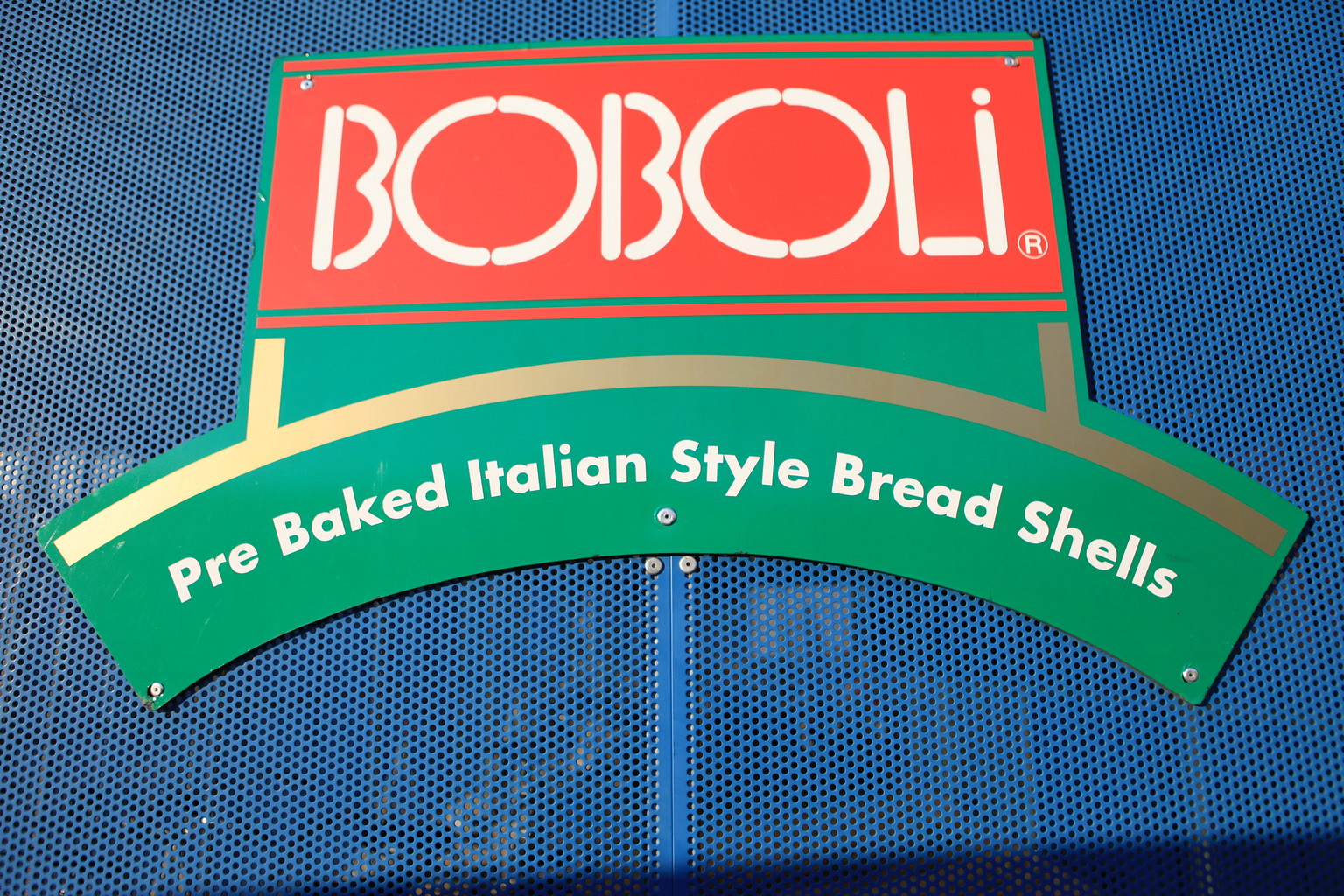The image features an outdoor sign mounted on a perforated blue metal gate, likely indicating the entrance to a Boboli bread factory or kitchen area. The sign itself is rectangular with a noodle-like shape on top, displaying "Boboli" in white text set against a red background with a green stripe surrounding it. Below this, the sign reads "pre-baked Italian style bread shells" in green text. The sign is affixed to the blue mesh gate using visible rivets, adding a functional touch to its vibrant, attention-grabbing design.